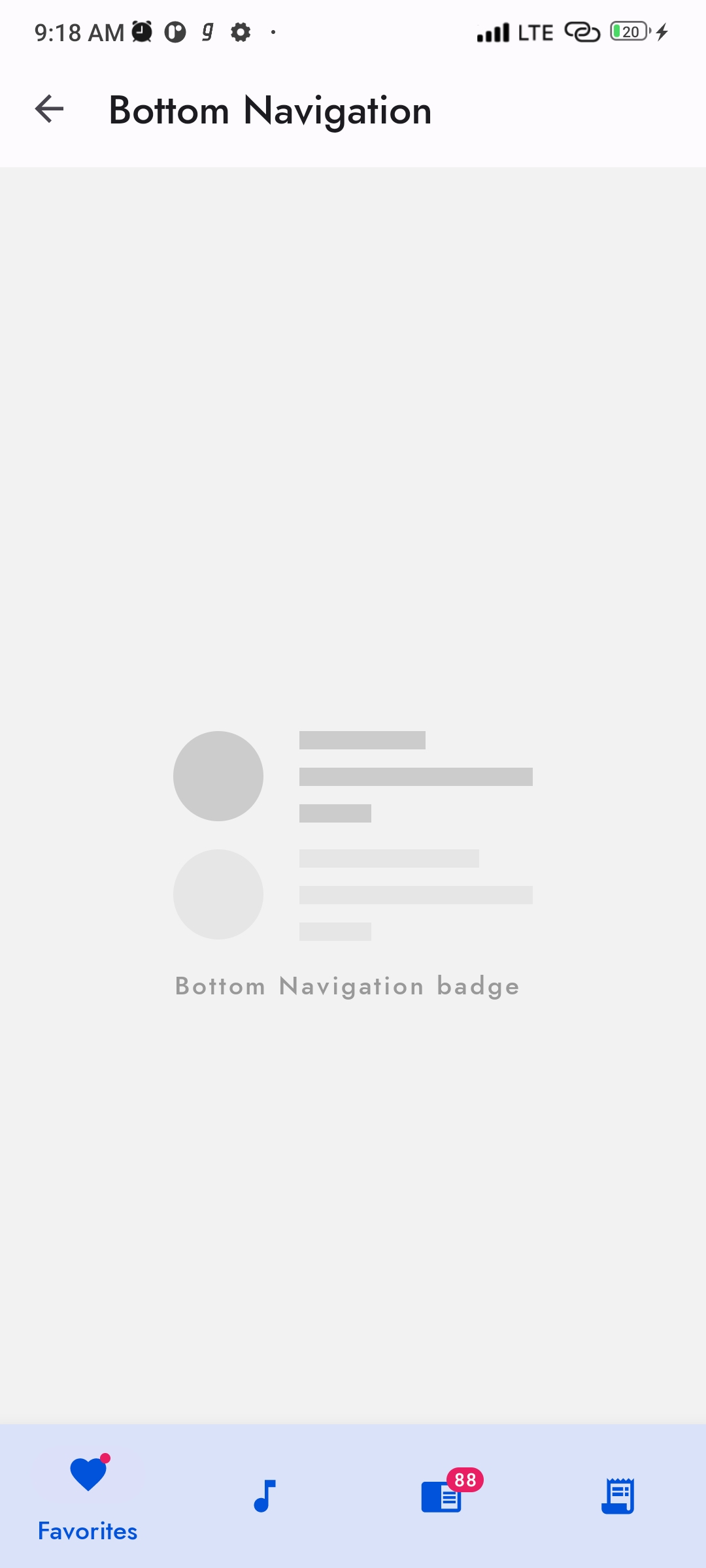The image is a screenshot from a mobile website. At the top of the image, there's a light gray background bar with several icons: the current time "9:18 AM" in black text, an alarm clock icon, a circle with an "R" inside, a lowercase "g," a gear icon, and a dot. On the right side of the bar, there are additional icons indicating cell signal strength, LTE connectivity, two connecting ovals, a battery icon showing 20% with a lightning bolt on its outline, and an arrow pointing to the left. Below this, the background transitions into a slightly darker gray. 

There is a circle in darker gray with three horizontal lines of varying lengths: a medium line, a long line, and a short line. Adjacent to this is a lighter gray circle also containing three horizontal lines of different lengths in the same sequence. These elements sit within a section labeled "Bottom Navigation Badge."

At the very bottom of the image, there is a blue banner featuring several icons and text labels: a heart icon labeled "Favorites," a music note, a square with text lines next to the number "88," and another small square with text lines, topped with a stylized graphic.